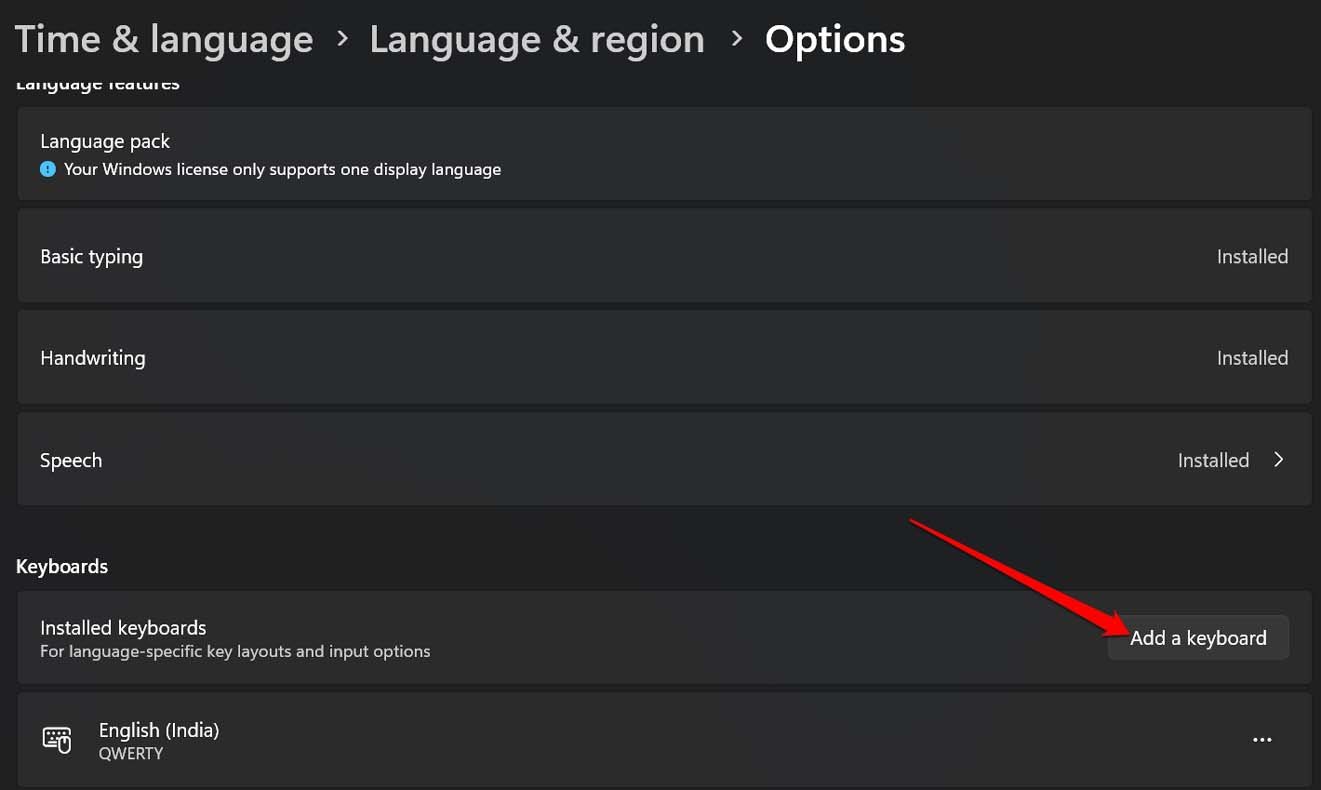In the photograph, there is a screenshot of a computer application with a black background displaying "Time & Language" in white text at the top. To the right, there is a right-pointing arrow next to the words "Language & Region," followed by another arrow pointing right next to "Options," also written in white.

Below, a section labeled "Language Features" is shown. At the top of this section, there is a blue exclamation mark with a message stating, "Your Windows license only supports one display language." Underneath, a box lists "Basic Typing" as installed. Another box shows "Handwriting" as installed, and yet another box indicates that "Speech" is installed, accompanied by an arrow to the right to access more options.

Farther down, there is a "Keyboards" section displaying the message, "Installed keyboards for language-specific key layouts and input options." A prominent red arrow points towards an option labeled "Add a keyboard." The final box in the screenshot shows the installed "English (India) QWERTY keyboard."